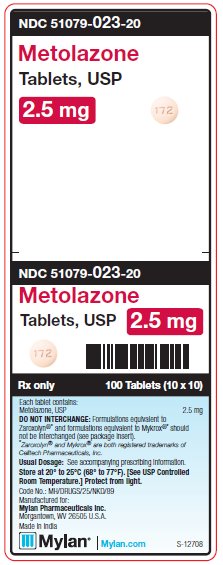In this image, the top section presents text in white on a black background, displaying "NDC 51079-0232-0." Beneath this, transitioning to a white background, the text changes to red, proclaiming "Metrolar Zone." Below that, in black text, it states "Tablet USP." Directly underneath is a red box with white text indicating "2.5 mg," thus describing the product as "Metrolar Zone Tablet USP 2.5 mg."

On the right side of the image is a depiction of a pink pill, marked with "172." Below the main section, in the center, another band of text written in white on a black background repeats, "NDC 51079-0232-0." Beneath this, it reiterates "Metrolar Zone Tablet USP 2.5 mg," and an identical pink pill image appears on the left side.

To the right is a black barcode. Below, the text specifies "Rx only" and "100 tablets (10 x 10)." Further down, there's a small, detailed description mentioning that each tablet contains specific ingredients, a caution to not interchange, and standard usage instructions, suggesting consulting the prescribing information. It also includes storage instructions, "Store at 20°C to 25°C (68°F to 77°F)." At the very bottom, "mylan.com" appears in blue, underlining the manufacturer's website.